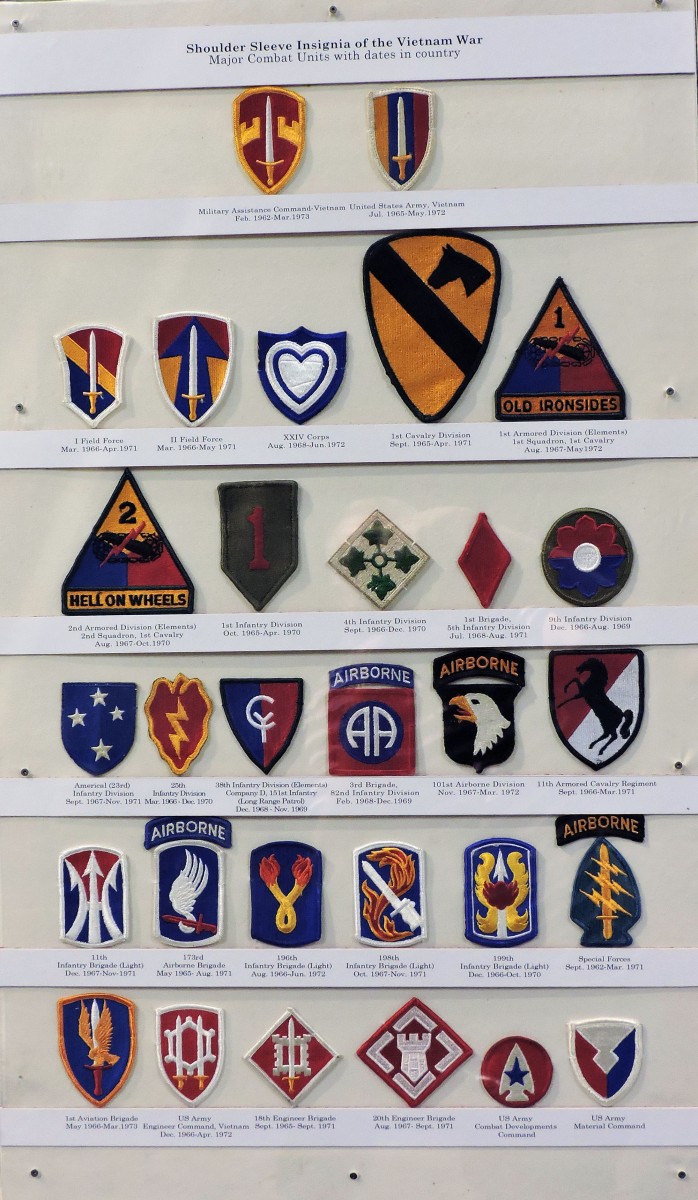This image features a meticulously arranged collection of military patches displayed against a white background. The display, seemingly framed and designed to be mounted on a wall, showcases 31 patches in total, organized into six rows with precise labeling beneath each patch. The top of the display is labeled "Shoulder Sleeve Insignia of the Vietnam War, Major Combat Units with Dates and Country," emphasizing its historical significance. 

The patches vary in shape and size, ranging from small to hand-sized, and are vibrantly colored in reds, oranges, yellows, and blues. The top row contains two patches, followed by five patches each on the second and third rows, six patches on the fourth row, seven on the fifth row, and six on the final row. Each patch represents different military units, identifiable by distinct insignias such as a golden eagle, an arrow spear with a blue star, horses, shields, and swords.

Prominent labels and specific terms include "Airborne," "Hell on Wheels," and "Old Ironsides," indicating different divisions and notable units. Alongside these, the design elements feature orange collars, red collars, blue collars, white and black horses, and yellow swords, further highlighting the diversity and the historical context of these badges. Each row is underlined by a narrow white strip of typed descriptions, likely detailing the patch's origin, associated unit, and the specific missions or honors from the Vietnam War period.